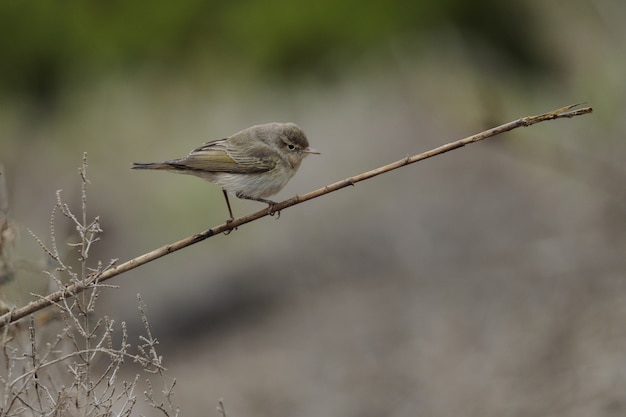This photograph captures a close-up scene of a small bird perched halfway up on a diagonal branch, which extends from the bottom left to the top right of the image. The scene is rendered in a muted palette of grays, browns, and tans, giving it a somewhat lifeless appearance. The background is completely out of focus, blurring any distinguishable features but hinting at variations in earthy tones and a patch of green.

On the bottom left of the image, thin twigs and foliage reach upward, adding to the composition. The bird, facing to the right, displays an intricate mix of colors: a primarily gray-brown body with a light gray belly, subtle greenish hues intermingled with darker feathers, and a touch of black on its tail. Its teeny, black eyes and bent legs contribute to its delicate form. Small details, such as the tiny white buds on the branches and the bird’s slight yellowish tint on the breast and wings, complete this serene yet detailed portrait of nature.